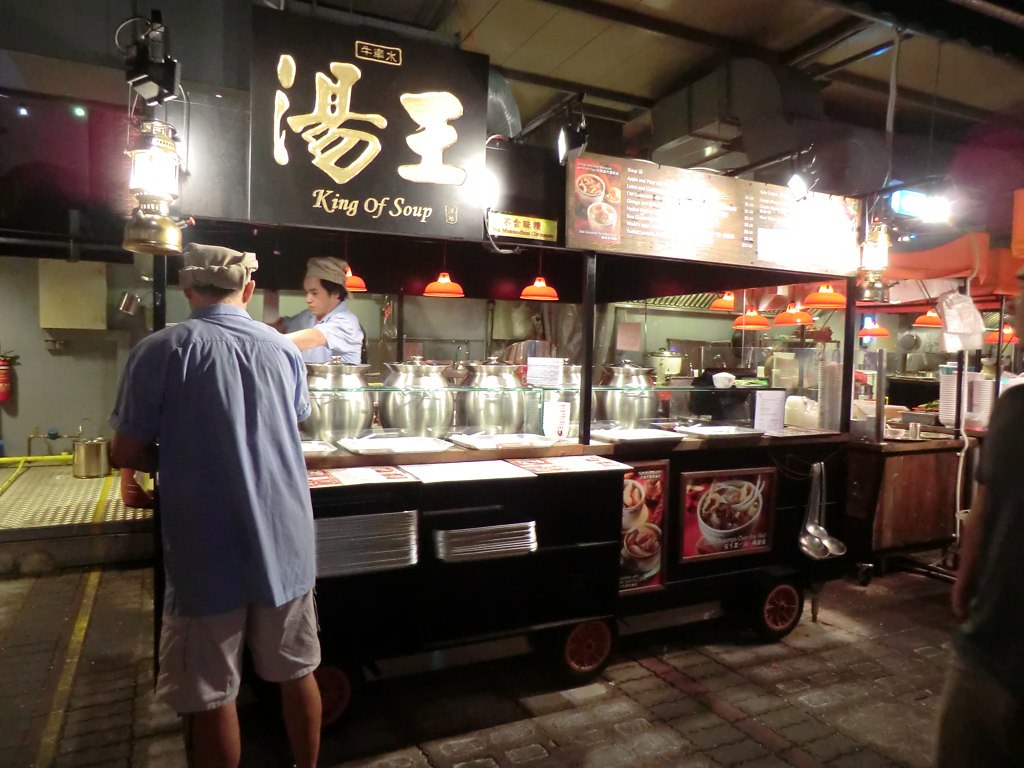The image depicts the interior of a restaurant that features multiple rolling carts. The main cart on the left showcases a sign with Chinese characters and the title "King of Soup" in gold on a black background. This cart has three large stainless steel soup pots with lids. A chef in a white hat and a blue shirt is busy behind the counter. To the right, another cart associated with the King of Soup has a menu, though it is unreadable due to glare from overhead lights. The restaurant's floor is made of brick, and there are metal ladles hanging from one of the carts. A man in khaki shorts and a blue shirt, possibly another employee, stands in the vicinity with a towel-like wrap around his head, suggesting he may be preparing for the day. The setup hints at a variety of soup offerings and a bustling workspace.